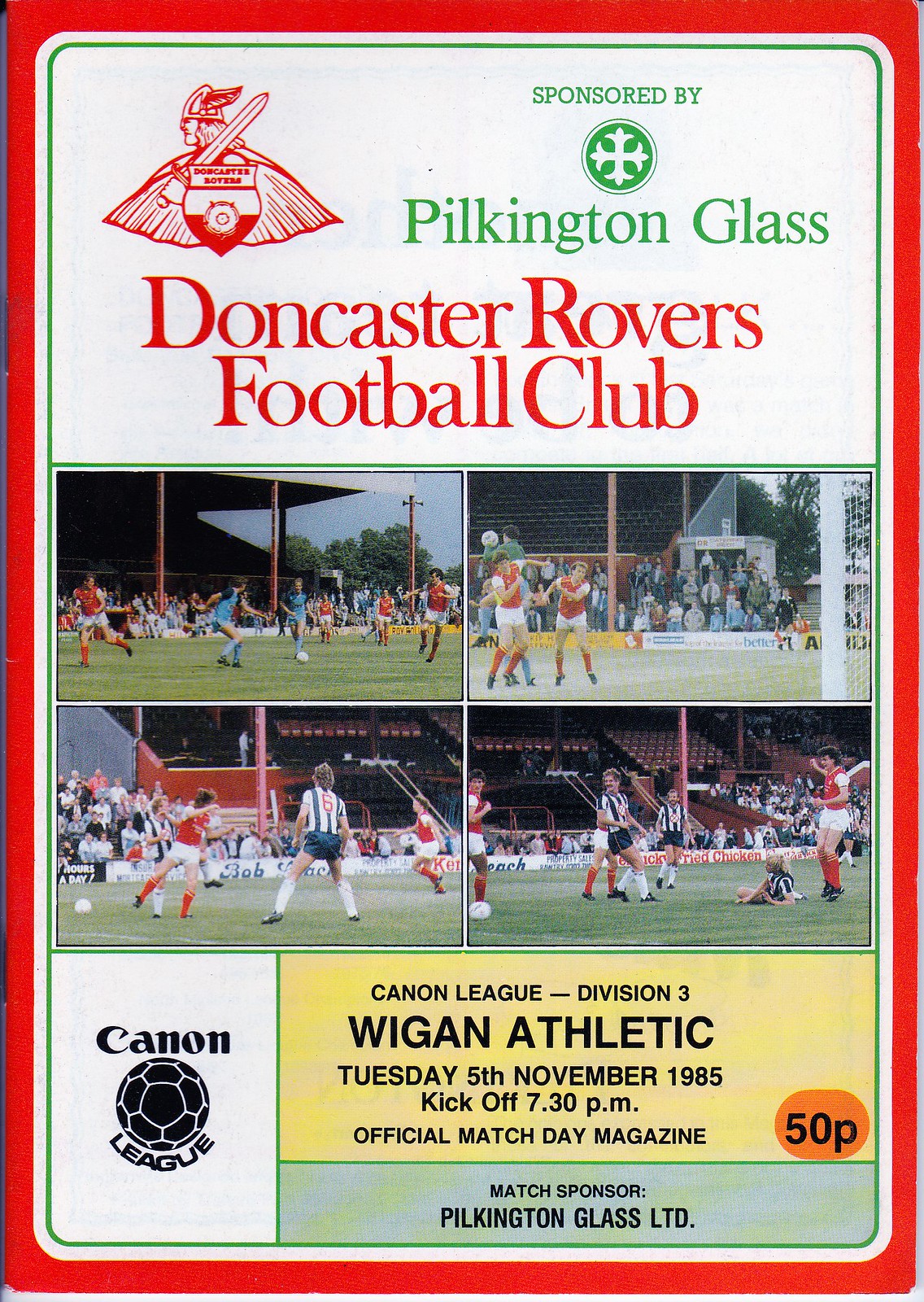The front cover of the soccer program for the Doncaster Rovers Football Club is primarily white with a red border, designed like a magazine. At the top left, there is a red logo of a Viking holding a sword and shield, next to green text that reads, "Sponsored by Pilkington Glass." Below this, in larger red font, it says, "Doncaster Rovers Football Club." The middle section of the cover features four images arranged in a 2x2 grid, showing players in action during soccer matches, with stadiums visible in the background. Players are seen wearing blue or red jerseys.

In the bottom third of the cover, on the left, there is a white box with black text that says, "Canon League" with a soccer ball in the middle. To the right, the cover is split into two sections. The top section has a yellow background with black text that reads, "Canon League, Division III, Wigan Athletic, Tuesday, 5th November 1985, kick-off 7.30 p.m., Official Match Day magazine." An adjacent orange box has "50p" in black font. Below this, a green area states, "Match Sponsor: Pilkington Glass LTD."